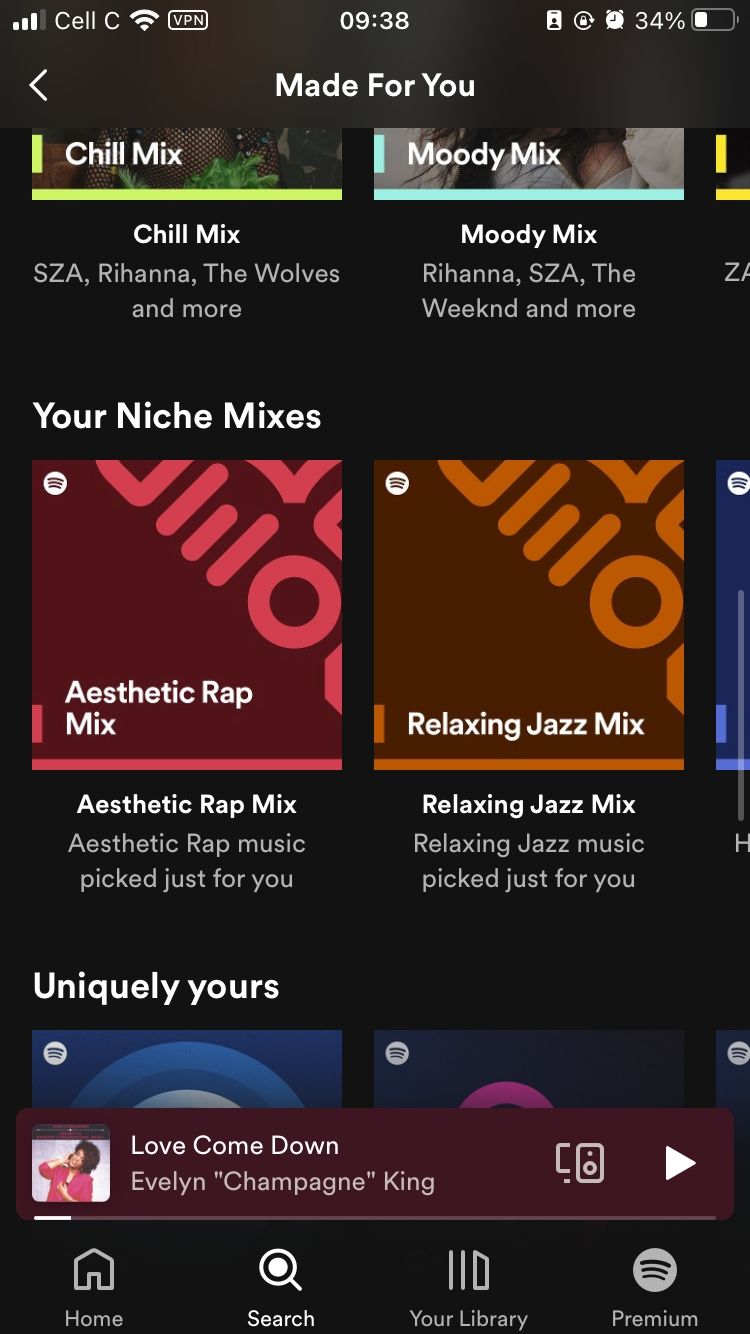This detailed description is based on a screenshot of a Spotify mobile interface. The current time displayed on the top taskbar is 9:38, and the battery status shows 34% remaining. Additional icons on the taskbar indicate that the device is using Cell C as the mobile network provider and is connected to a VPN.

The main interface displays a variety of Spotify playlists under different categories. The top bar of the app reads "Made for You," and features a back arrow on the left for navigation. The playlist section is partially cut off, hiding some of the playlist thumbnails at the bottom edge.

The first row features playlists titled:
- "Chill Mix," which includes artists like SZA, Rihanna, The Wolves, and more.
- "Moody Mix," featuring Rihanna, SZA, The Weeknd, and more.
- Another playlist on the right is only partially visible.

Below this, the header "Your Niche Mixes" presents:
- "Aesthetic Rap Mix," described as "Aesthetic rap music picked just for you."
- "Relaxing Jazz Mix," offering "Relaxing jazz music picked just for you."
- A third mix on the right is also partially cut off.

The third section, titled "Uniquely Yours," is also visible but partially cut off, showing a couple of playlist or album covers.

At the bottom of the screen, the currently playing track is "Love Come Down" by Evelyn "Champagne" King. The bottom navigation bar includes icons for Home, Search, Your Library, and Premium features, accompanied by a small speaker icon, and a play button.